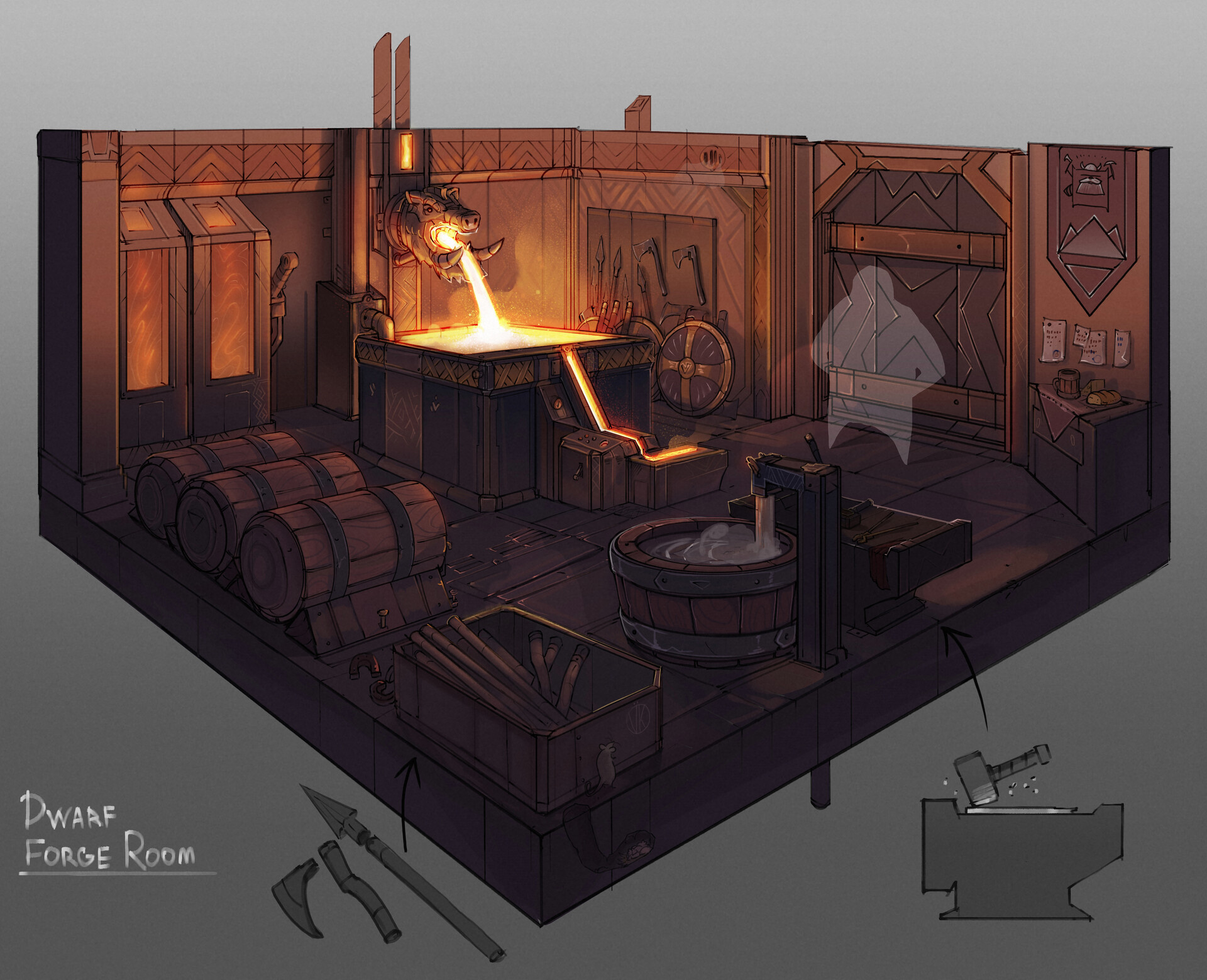The illustration, possibly a computer-generated concept art of a dwarf forge room, predominantly features brown hues with a silverish-gray background, giving it a metallic industrial feel. The scene is set within a square cutout room furnished with wooden paneling. In the lower left-hand side, there are three large wooden barrels or casks. Nearby, a dragon-shaped figurehead on the wall spews fiery molten metal into a substantial metal vat, which overflows into a smaller container below it. Adjacent to this setup is a large wooden tub filled with water, fed by a stylized animal-head faucet emanating directly from the floor.

Tools associated with metalwork, including various forge tools, an anvil, and a hammer poised as if in motion, are scattered throughout the room. Weapons like axes, shields, and spearheads adorn the corners, emphasizing the space's utilitarian purpose. On the far wall, there's a door, and next to it is the faint outline of a dwarf figure, suggesting someone standing guard or at work. The words "Dwarf Forge Room" are inscribed in white script in the bottom left corner of the image, adding a finishing touch to this detailed depiction of a bustling forge setting.